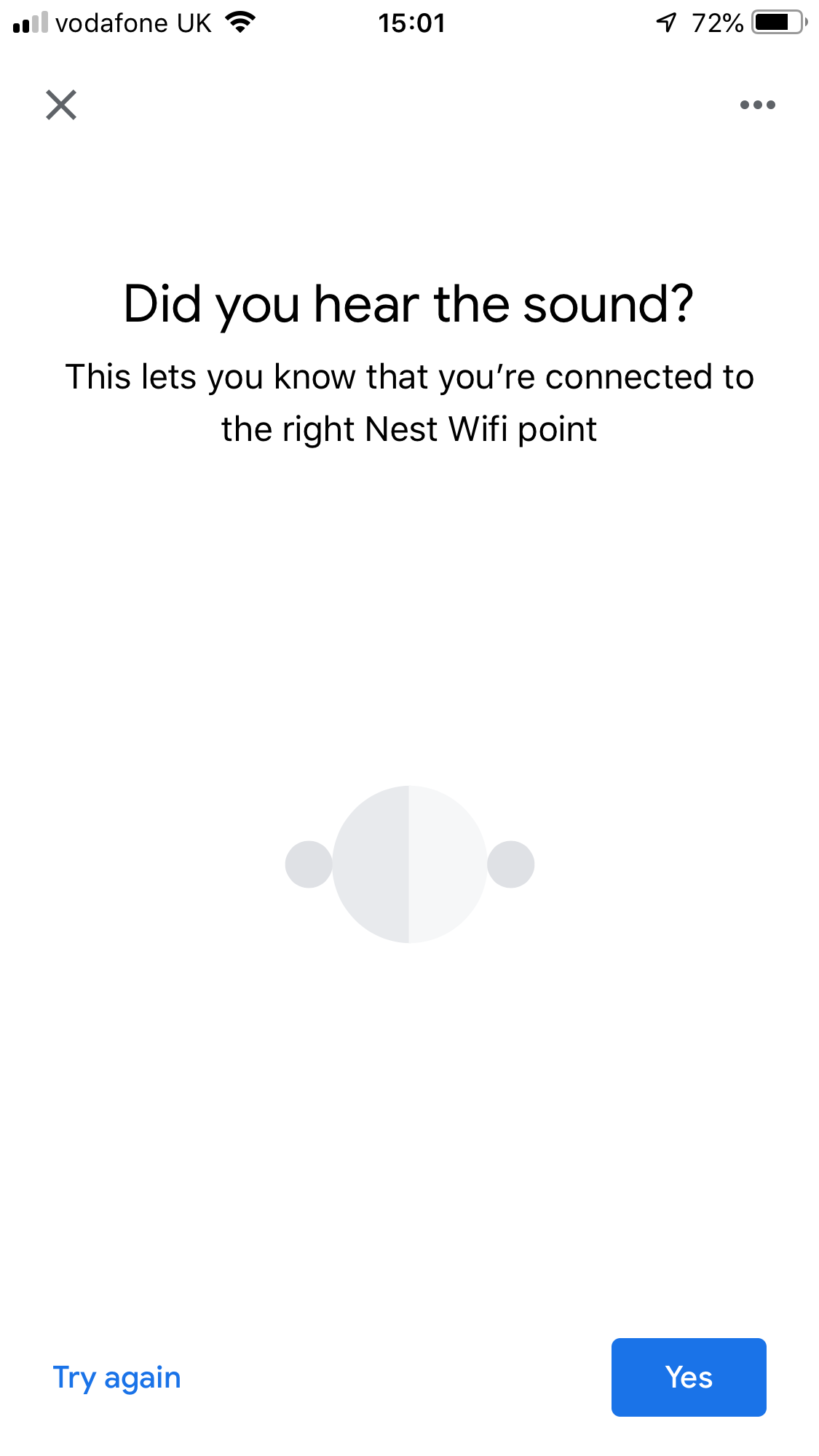The image features a white background with several interface elements. In the top-left corner, it displays "Vodafone UK" alongside "1501", with an arrow pointing up and to the right. The battery indicator shows 72% charged. Adjacent to these elements, there is an 'X' in the left corner and three vertical dots on the right.

A prominent text reads "Did you hear the sound?" that confirms the connection to the correct Nest Wi-Fi point. Centrally positioned, there's a large circle divided into two halves: one dark gray and the other light gray, each accompanied by a smaller circle in dark gray.

At the bottom of the screen, there are two interactive buttons: one stating "Try Again" in blue text on the left, and a blue "Yes" button on the right.

The overall layout is designed to confirm the Wi-Fi setup process, guiding the user through steps with clear prompts and interactive options.